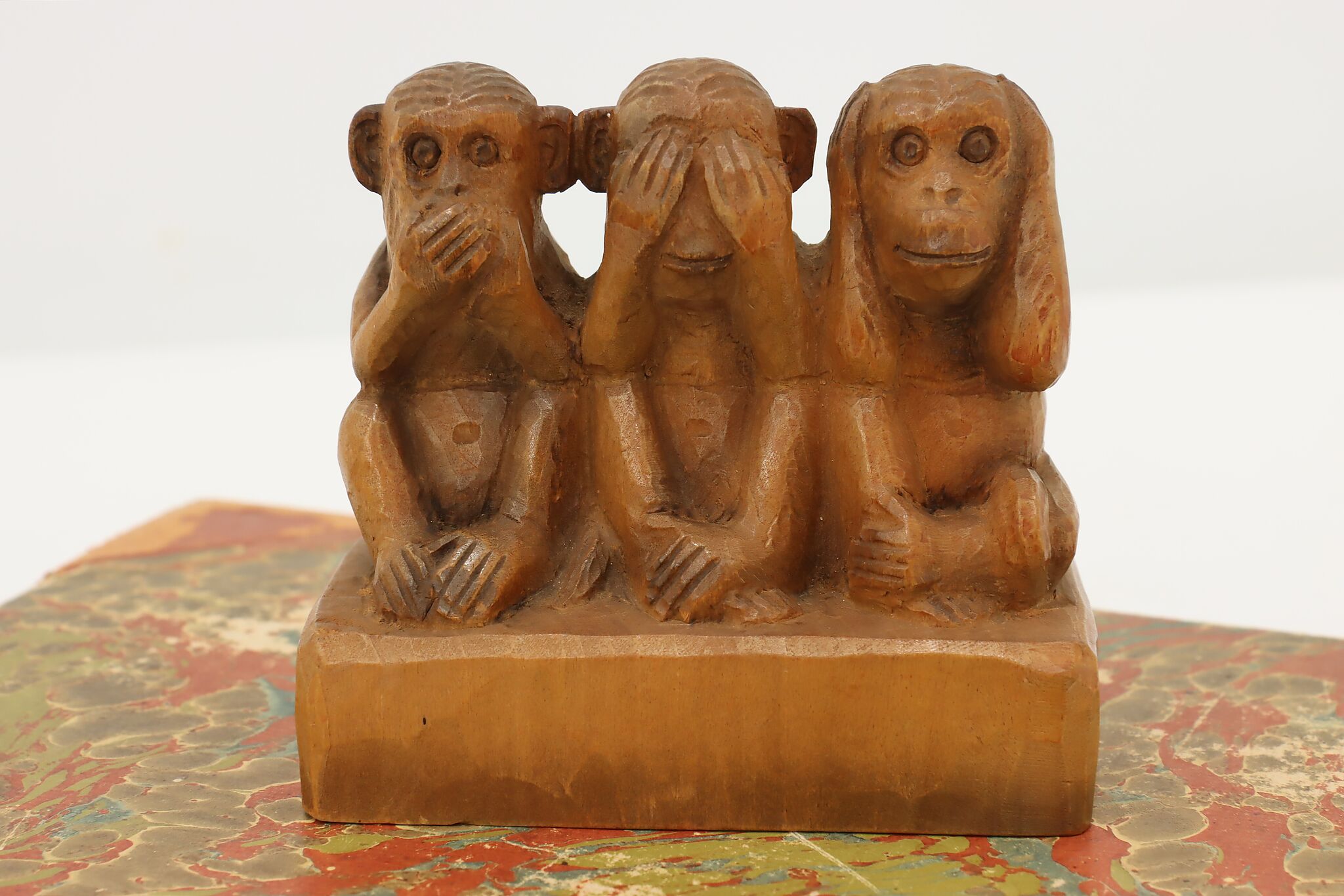The image is a detailed color photograph of a wooden sculpture featuring three small monkeys arranged in a row. Each monkey embodies a segment of the well-known adage "see no evil, hear no evil, speak no evil." The sculpture, meticulously carved from light brown wood, shows the textured grain and craftsmanship. The first monkey on the left covers its mouth with both hands, the middle monkey covers its eyes, and the last one on the right covers its ears. All three figures, with their feet folded over each other, emanate a sense of mischief. They are connected as a single piece, sitting on a rectangular wooden platform. The sculpture rests on a table that appears worn, with remnants of red or blue paint now bubbled and blotched, suggesting age or exposure to heat. The background of the image is stark white, highlighting the rich details and artistic expression of the piece.